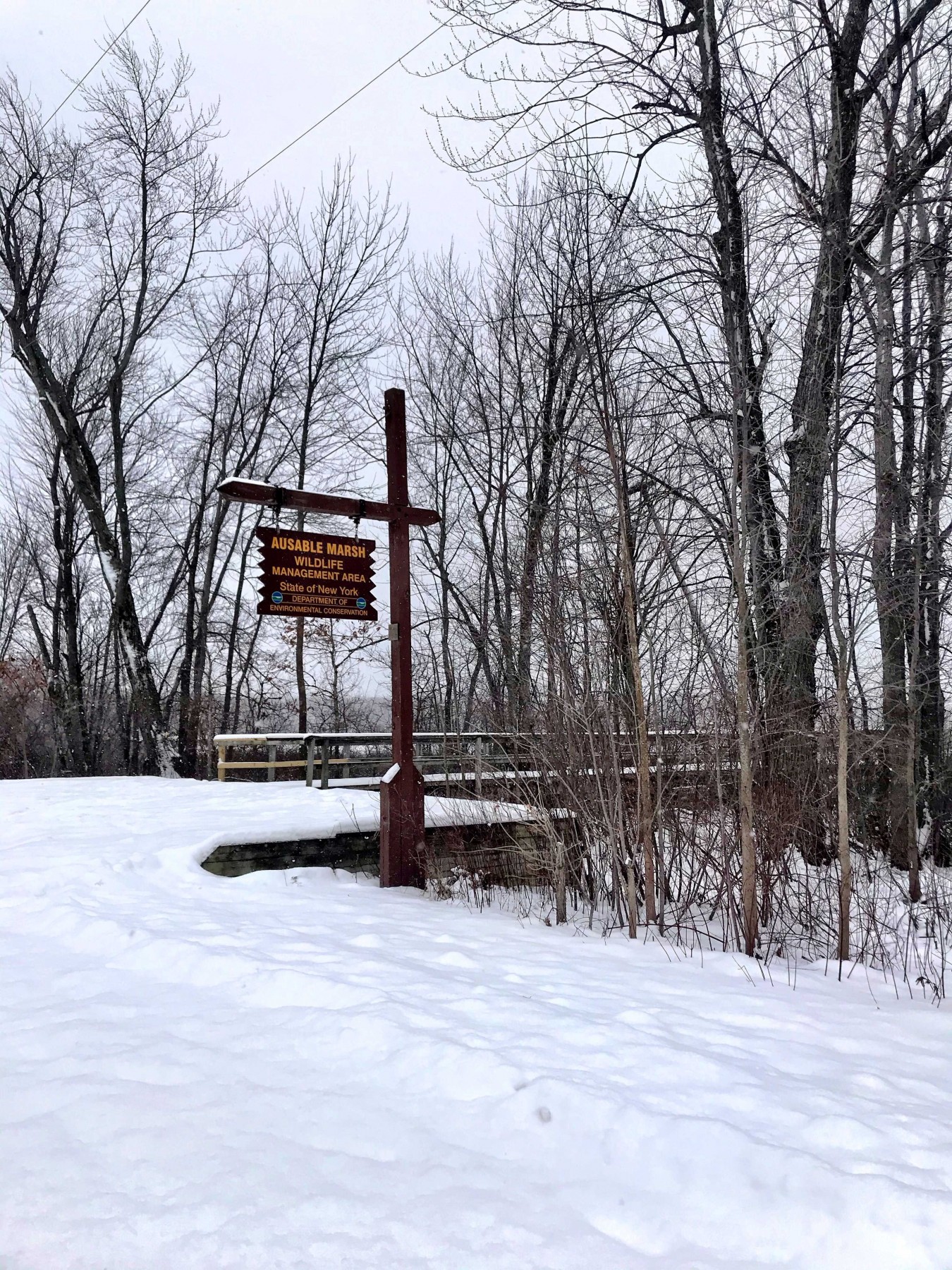This photorealistic image captures a serene winter scene at the entrance to the Ossable Marsh Wildlife Management Area in the State of New York. The landscape is blanketed with three inches of snow, covering the ground uniformly under a gray, overcast sky. The trees in the background are bare, their branches standing stark and leafless against the muted sky. Located in the snowy foreground is a prominent, dark, wooden, T-shaped sign hanging by chains from a crosshatched pole. The sign features yellow writing, partially readable, with the words "Ossable Marsh Wildlife Management Area" clearly visible. Behind the sign, a snow-covered bridge extends diagonally from the left-hand side to the fading back right-hand side of the picture, hinting at a pathway that continues deeper into the wooded area. Power lines can be seen traversing overhead. The scene is tranquil and devoid of active snowfall, evoking the quiet stillness of a winter day.